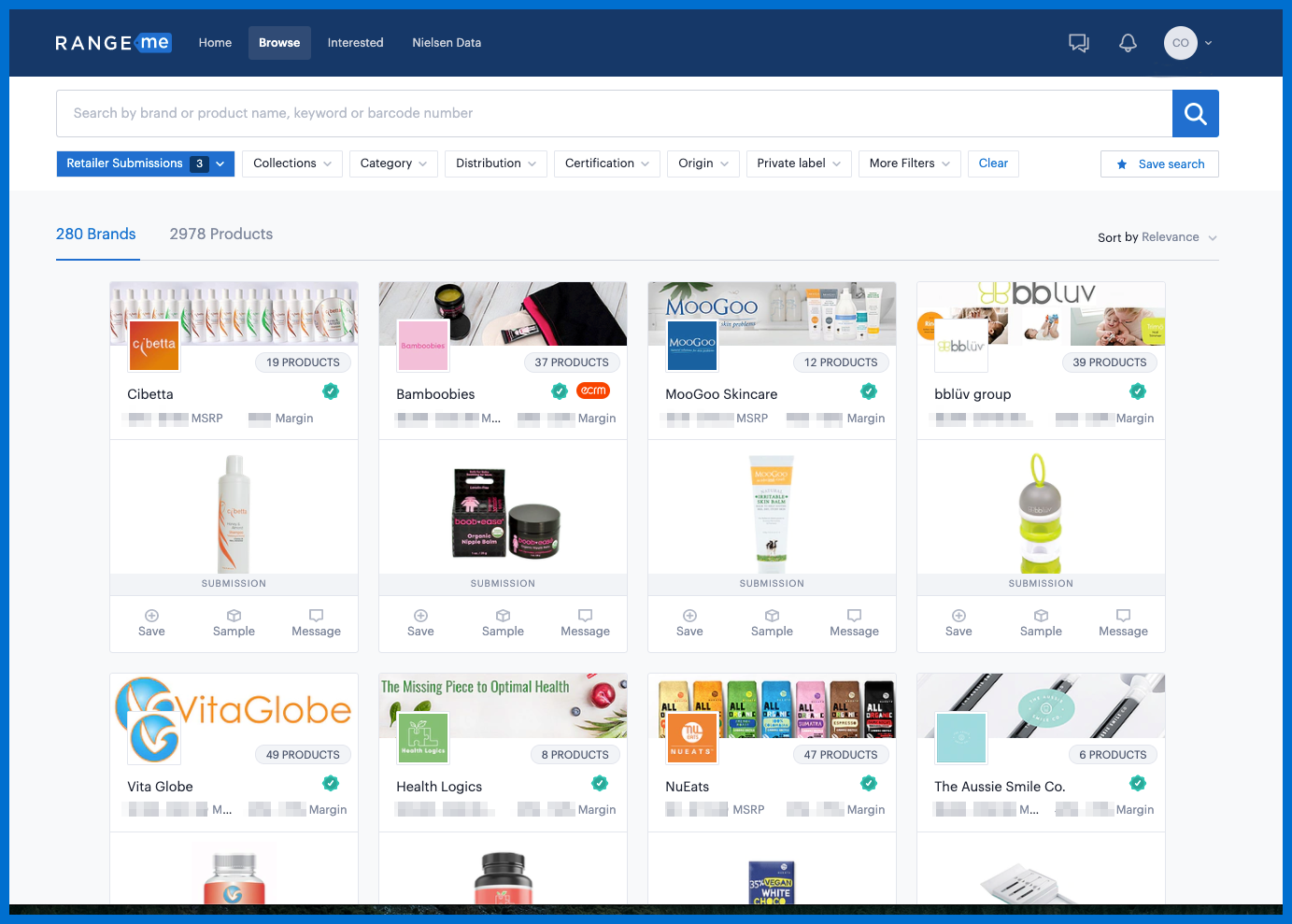This image is a screenshot of a webpage displaying a selection of products, arranged in a grid format. The grid consists of two rows, with each row containing four rectangular product display sections. In the first row:

1. The first rectangle depicts what appears to be a bottle of conditioner.
2. The second rectangle shows a circular jar, possibly a hair product, with a lid that can be opened.
3. The third rectangle is labeled "Moogoo Skincare" and features a bottle with a screw-top circular cap.
4. The fourth rectangle is less clear due to a small, blurry image but seems to depict a circular tube of some sort.

The second row of products is partially obscured, revealing only the top portions of the products, making them difficult to identify.

Above each product representation, there is information about the seller, including the number of products they offer and their ratings. The background of the website is grey, and a search bar is prominently positioned at the top of the page, featuring a blue and white search icon. 

Users can filter the products using various options such as collection, category, distribution, certification, origin, and private label, among other filters. The top of the webpage features a navy blue header with the site name "Range Me" and navigation buttons labeled Home, Browse, Interested, and an unreadable fourth option.